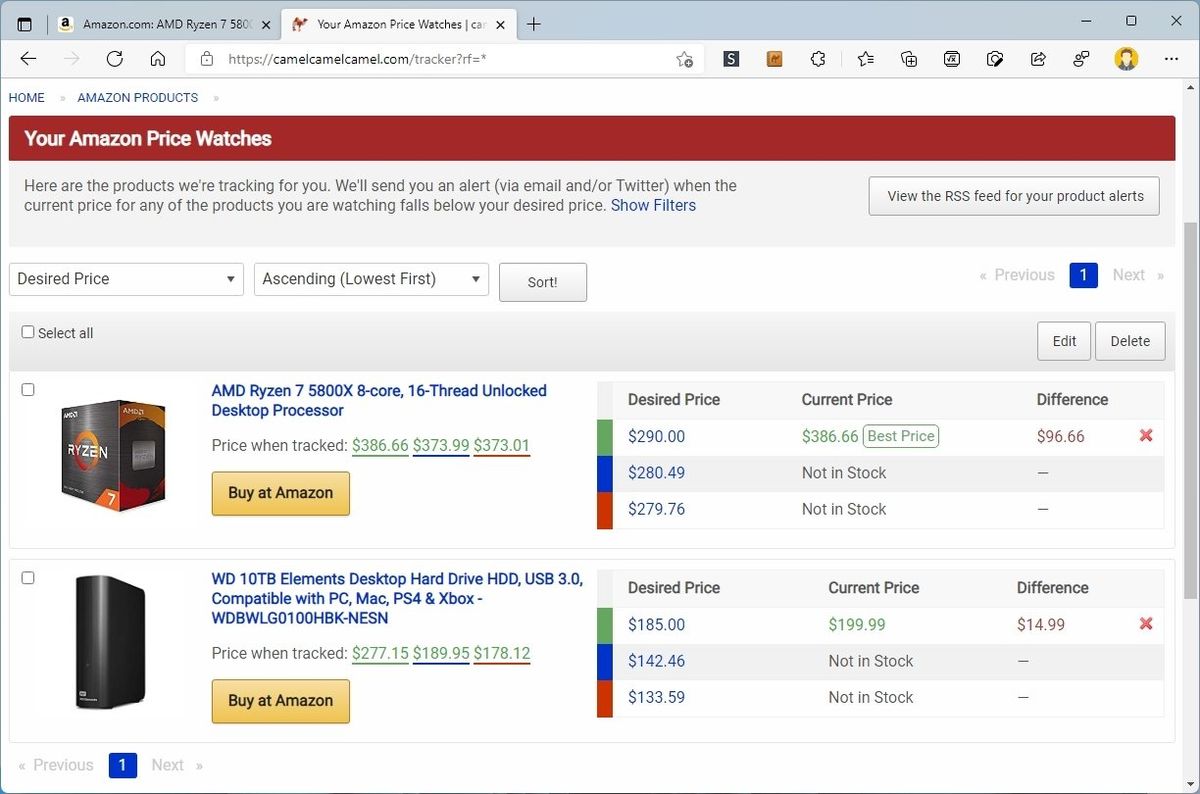The interface displayed on the screen shows a web browser with two open Amazon tabs, featuring the Amazon Price Watches website. At the top left corner, "Home Amazon Products" is clearly labeled. Below this, a prominent red strip carries the text "Your Amazon Price Watches" in white.

Beneath the header, a section outlines the service details: "Here are the products we're tracking for you. We'll send you an alert via email and/or Twitter when the current price of any of the products you are watching falls below your desired price." On the left side, a blue link labeled "Show Filters" is visible.

On the right side of the page, a gray-bordered box displays options for viewing the RSS feed for product alerts in gray font. Below this, there is an option labeled "Desired Price," which includes a dropdown menu for sorting with "Ascending lowest first." Next to this is a gray "Sort" button.

Navigational elements include a "Previous" button with a white numeral "1" inside a blue box on the left, and a "Next" button in gray on the right. Below these buttons, a "Select All" checkbox is present but not marked.

The list of tracked items begins with two examples. The first item is the "AMD Ryzen 7 5800X 8-Core 16-Thread Unlocked Desktop Processor." The price details for this item show:

- Tracked Price: $386.66
- Previous Prices: $373.99, $373.01
- Desired Price: $290.00
- Current Price: $386.66

The second item's desired and current price are listed as $280.49, but no further details are provided.

This detailed overview vividly captures the function and layout of the Amazon Price Watches website.